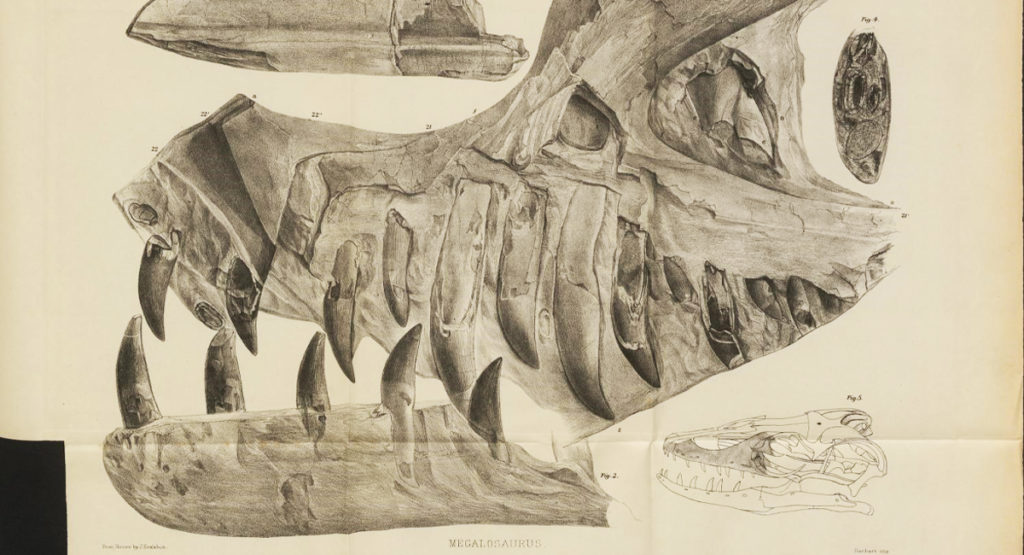The image features a detailed depiction of a fossilized dinosaur head, set against a cream-colored background. The dinosaur is facing left, with its mouth wide open revealing an array of long, dark black fangs. These fangs, some pointing upwards and others downwards, can be seen stretching both into the upper and lower jaws, displaying the bone structure prominently. The eye socket, positioned just below the center of the image, appears covered with an oval shape originating from the left. Small, unreadable numbers line the muzzle, which curves downwards to the center before ascending to the upper left corner and then descending steeply towards the left side.

In the very bottom left corner, a small black rectangle can be seen, while at the bottom right, there's a fine-lined sketch of the same creature, labeled “FIG5”. Above this sketch, there is some gray, blurry text that seems to spell "V-E-G-A-L-O-A-R-U-S". The upper right corner of the image also features a dark oval with black patches, above which a similarly unreadable “FIG5” appears. Evident in the drawing is the presence of a horn-like structure above the eye orbit, and near the top left of the skull, an isolated, partially cut-off pointy object, possibly one of the fangs, is visible.